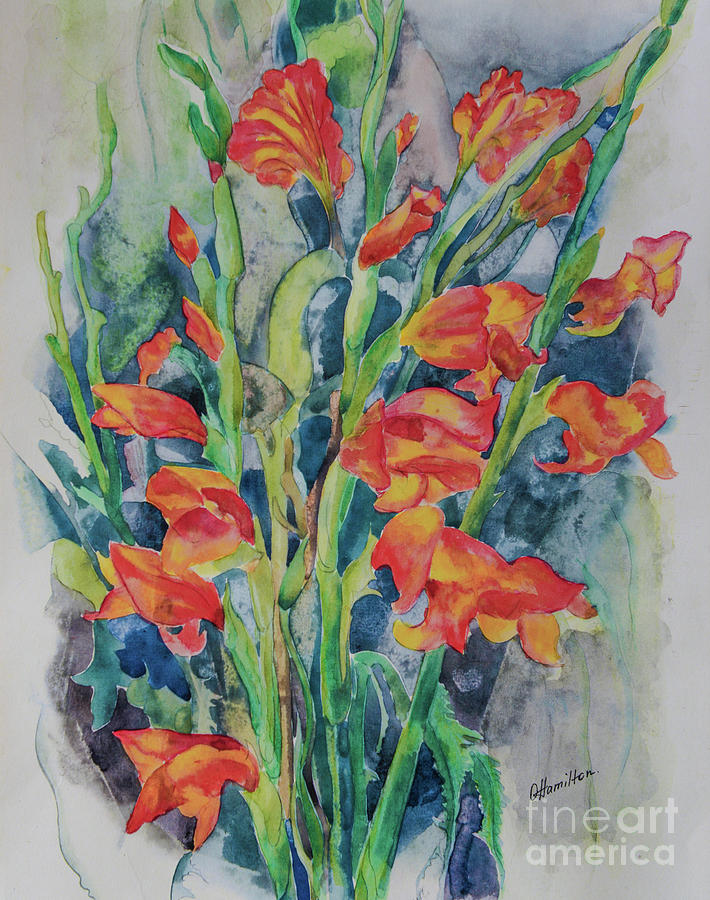This detailed watercolor painting depicts an array of flowers characterized by long, green stems sprawling across the lower section and jutting in various directions. The flowers, vibrant hues of orange and red reminiscent of snapdragons, are in various stages of bloom—some fully open, others just budding or half-open. Not all the stems culminate in flowers; some are bare, adding to the natural, varied appearance of the scene. The background features a blend of gray with darker black and blue areas, lending depth to the overall composition. The painting is signed "G. Hamilton" in cursive at the bottom right corner, with "Fine Art America" printed in lowercase white text superimposed on the gray background.